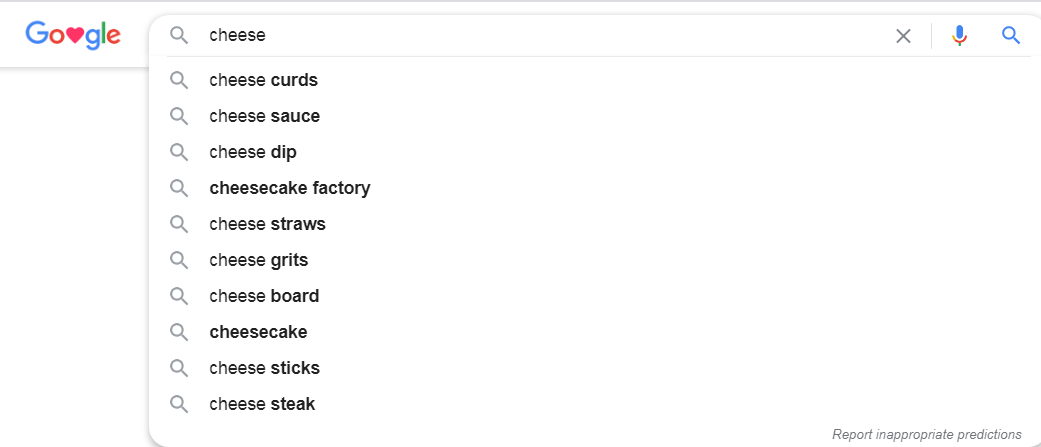The image depicts a Google search page with the word "cheese" typed into the search bar. The familiar Google logo is displayed prominently at the top, with the letters "G," "O," "O," "G," "L," and "E" in blue, red, yellow, and green, respectively. Of note, the second "O" is stylized as a heart.

In the search bar, the word "cheese" is written in black text. Below this, a dropdown list of autocomplete suggestions is visible:

1. Cheese Curds
2. Cheese Sauce
3. Cheese Dip
4. Cheesecake Factory
5. Cheese Straws
6. Cheese Grits
7. Cheese Board
8. Cheesecake
9. Cheese Sticks
10. Cheese Steak

Each suggestion is accompanied by a small gray magnifying glass icon to the left. On the right side of the search bar, there are additional interface elements: a gray "X" to clear the search input, a microphone icon in red, blue, and gray for voice search, and a blue magnifying glass to initiate the search.

At the bottom right corner of the dropdown, the text "Report Inappropriate Predictions" appears in gray. The background of the page is a clean white, emphasizing the simplicity of the Google search interface. The overall color scheme includes shades of blue, red, orange, green, gray, black, and white.